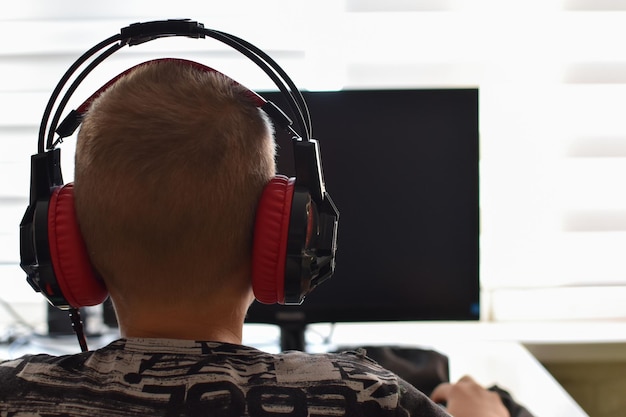In the image, a young man with short, closely cropped light brown hair is seated at a desk, intently focusing on a black, unlit computer monitor in front of him. The setting appears to be his room, judging by the basic furnishings and personal atmosphere. Behind the monitor, a window with white curtains partially drawn permits a stream of daylight that backlights both the monitor and the individual, giving them an almost silhouette effect. He is wearing a black and gray or possibly black and white t-shirt, which features some indistinguishable text or numbers—maybe a design or year like "1993."

The man is equipped with a large set of wired headphones, predominantly black but distinguished by vibrant red ear cups and a red strap that touches the top of his head; these headphones are essential to his setup. His right hand is placed on a computer mouse, ready to interact with the desktop facing him. Despite the backlighting, these details merge to paint a vivid picture of a focused gamer in his personal space.